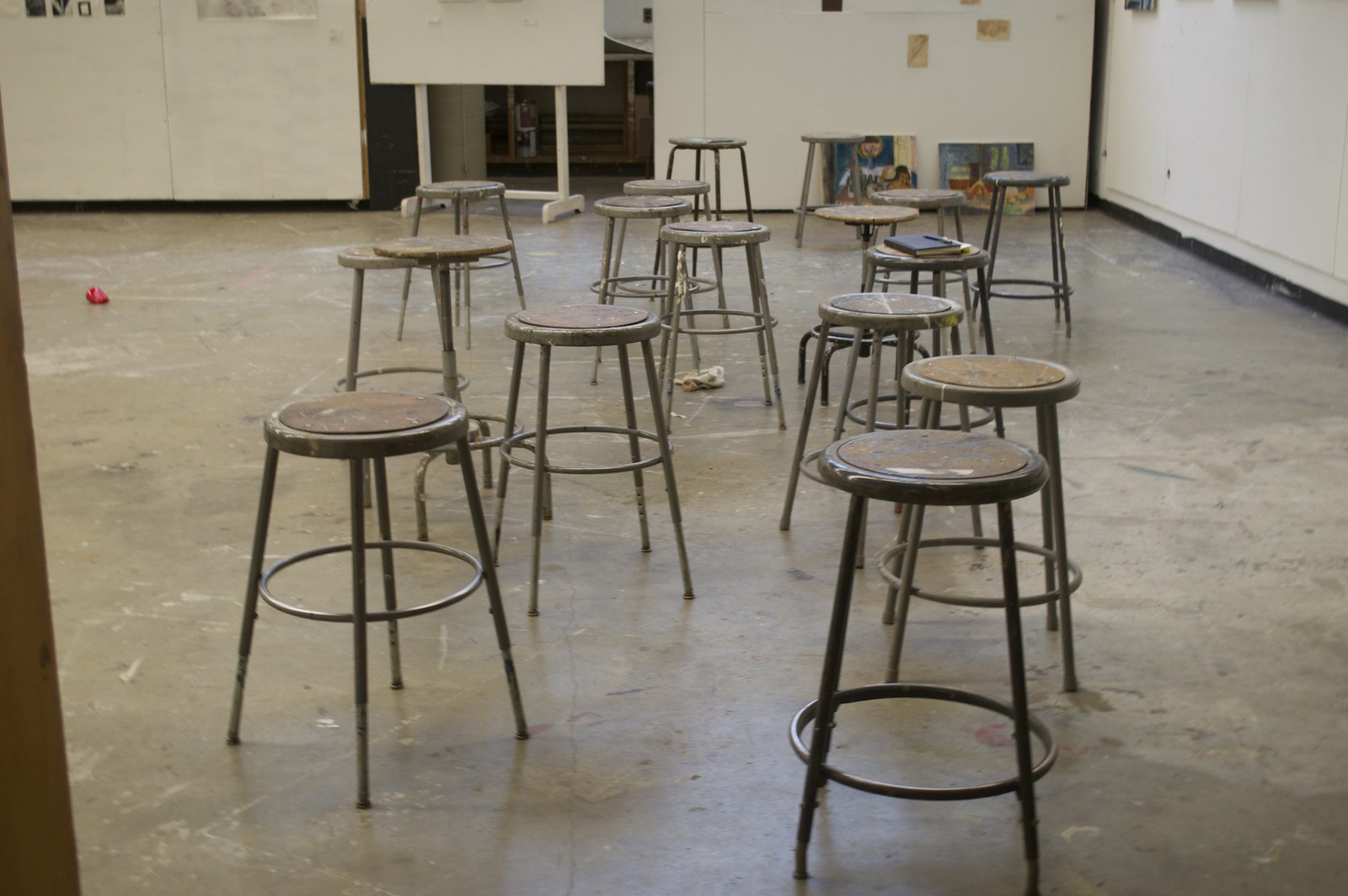The image depicts a large room with white walls adorned with several black-and-white photographs and a few paintings leaning against the bottom of the wall. At the center are approximately 15 to 20 round metal stools with legs that spread outward from the top, all colored in dark grey and appearing very old. These stools, along with a stray black book resting on one of them, sit on a very grey and worn-down concrete floor marked with white and black streaks and swirls of grey and brown. Against one wall, there is a large whiteboard mounted on a white base that stands prominently, resembling a posting area but entirely blank. In the background, a large doorway opens up to reveal a glimpse of another building outside, while a small red toy car lies on the floor inside, resembling a piece of discarded trash.